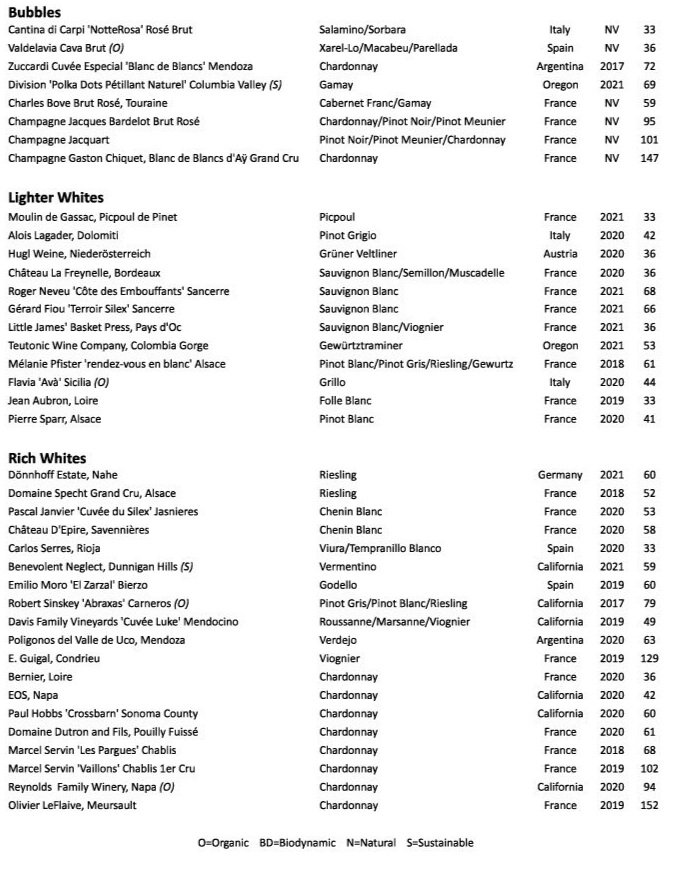The black-and-white photograph features a detailed wine list menu, meticulously categorized into three sections: Bubbles, Lighter Whites, and Rich Whites. Each of these sections is further divided into multiple columns, offering a comprehensive overview of the available wines. The leftmost column displays the name of the wine, followed by the type of grape used in the center column (such as Chardonnay). The third column specifies the region of origin, which includes a diverse range of countries like France, Italy, Spain, Argentina, Oregon, and Germany. The fourth column lists the year of production when available, with years such as 2021, 2020, and 2018. The fifth column contains unlabeled numbers ranging from 50 to 152, whose purpose remains unclear. The bottom of the menu includes a key that decodes several symbols: O for organic, BD for biodynamic, N for natural, and S for sustainable. The Bubbles section offers ten options, featuring various types of sparkling wines from countries like Italy, Spain, Argentina, Oregon, and France. The Lighter Whites section, with over ten selections, predominantly features wines from France but also includes options from Italy and Austria. The Rich Whites section is the most extensive, including wines mainly from France, with additional options from Germany, Spain, California, and Argentina.